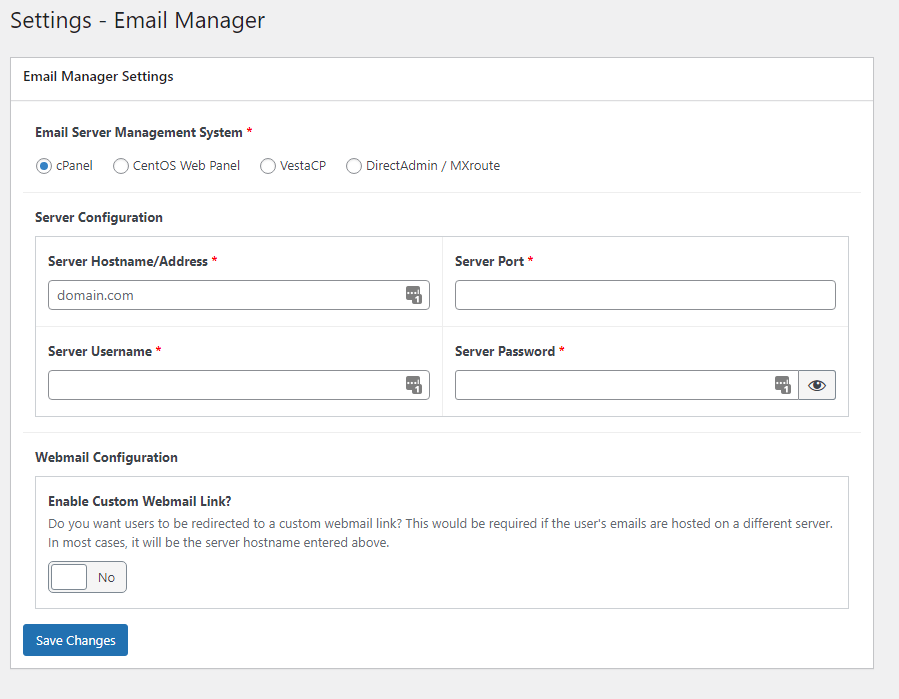A detailed image description for the given voice caption could be:

"The image displays a 'Settings' window titled 'Email Manager.' It appears to be part of an email client or server management application. At the top, the section header reads 'Email Server Management System.' This section offers options for selecting an email management platform, specifically listing 'cPanel, CentOS, Vesta, DirectAdmin, and MXroute.' In this instance, 'cPanel,' the first option, has been selected.

Below the platform selection, there are fields for 'Server Configuration,' where users must input details such as 'Hostname and Address,' 'Server Ports,' 'Username,' and 'Server Password.' Further down, there is a subsection labeled 'Webmail Configuration.' This section includes a toggle to 'Enable Custom Webmail Link,' accompanied by a question: 'Do you want users to be redirected to a custom webmail link?' It explains that this may be necessary if users’ emails are hosted on a different server, and suggests that the custom webmail link will usually be the server hostname entered previously. Currently, the toggle is set to 'No.'

At the bottom of the window, there is a prominent blue 'Save Changes' button. The overall layout is clean with a white background and predominantly black text, typical of many settings interfaces. This image seems to showcase the steps an administrator might follow to set up an email server using specific server management software."